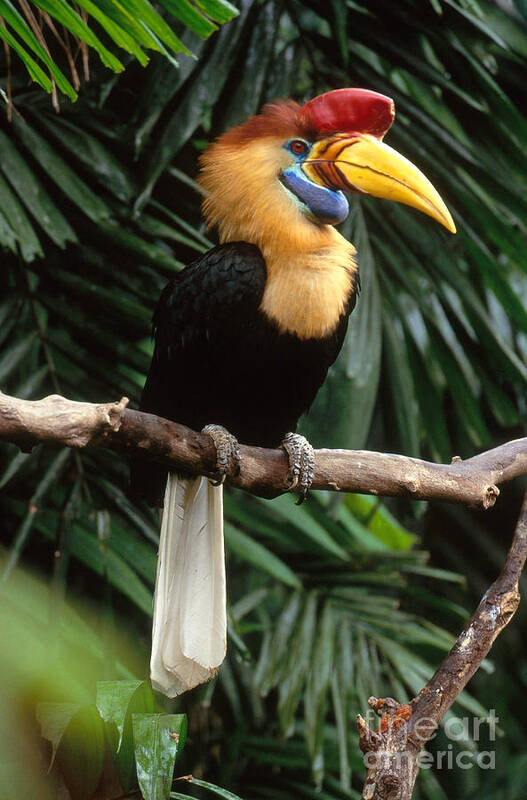This rectangular photograph captures a vibrant tropical bird, perched prominently on a branch against a lush backdrop of palm foliage. The bird's striking features include a long, yellow beak with an orange stripe near its face, a prominent red mound of skin or flesh atop the beak, and small, orange eyes with black pupils. The bird's head and face are adorned with vivid red and yellow feathers, transitioning to a black-feathered body and culminating in a white-feathered tail. The detailed, photorealistic image reveals the bird in profile, showcasing its distinctive coloration and intricate feather patterns. In the lower right-hand corner, a faint watermark reads, "Fine Art America" accompanied by a copyright symbol, subtly blending into the natural scene.